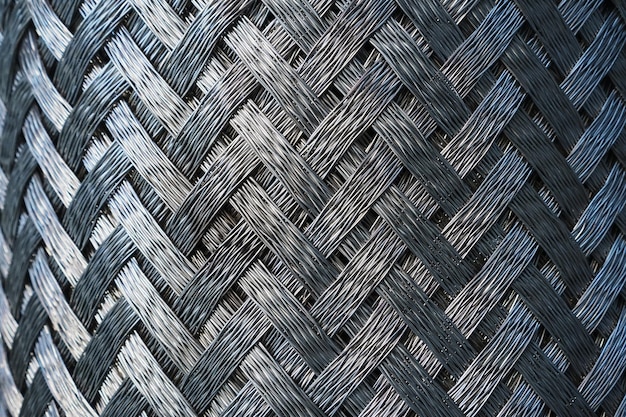This image is a detailed, up-close photo of a finely woven basket weave pattern, featuring tightly interlaced fibers that are black and grey with a reflective sheen concentrated on the left-hand side. The material, potentially plastic or finely-woven metal such as aluminum, is composed of numerous fibrous strands arranged into uniform, flat strips. These strips follow a meticulously consistent pattern, alternating by going over two strands and under one. The texture appears very tight and intricately woven, suggesting high precision, and the entire weave fills the frame of the image.